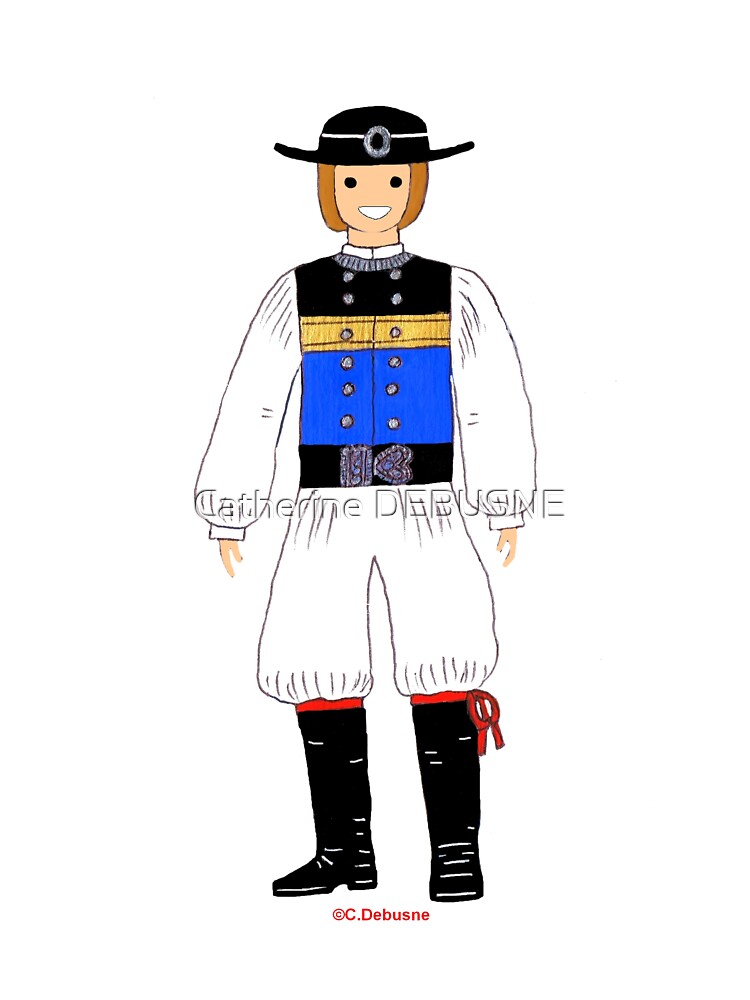This is an illustration of a cartoonish character, styled almost like a doll, bearing the printed name "Catherine Debusney" across the middle, with the copyright "C. Debusney" at the bottom. The character appears to be a long-haired person, potentially a man, with medium Caucasian skin tone and distinctive facial features including two simple eyes, no nose, and a white, upside-down triangle-shaped mouth. The hair is brownish-orange and reaches down to the chin. The individual is adorned in historical-looking attire resembling a pilgrim outfit. They sport a black bowler-style hat featuring a white stripe and a circular mark or buckle at the front. Their clothing comprises a white tunic and pants, which are puffy like breeches, topped with a multicolored vest that includes black, yellow, and blue sections along with two columns of buttons. Completing the ensemble are knee-high black boots with red ties just below the knees.